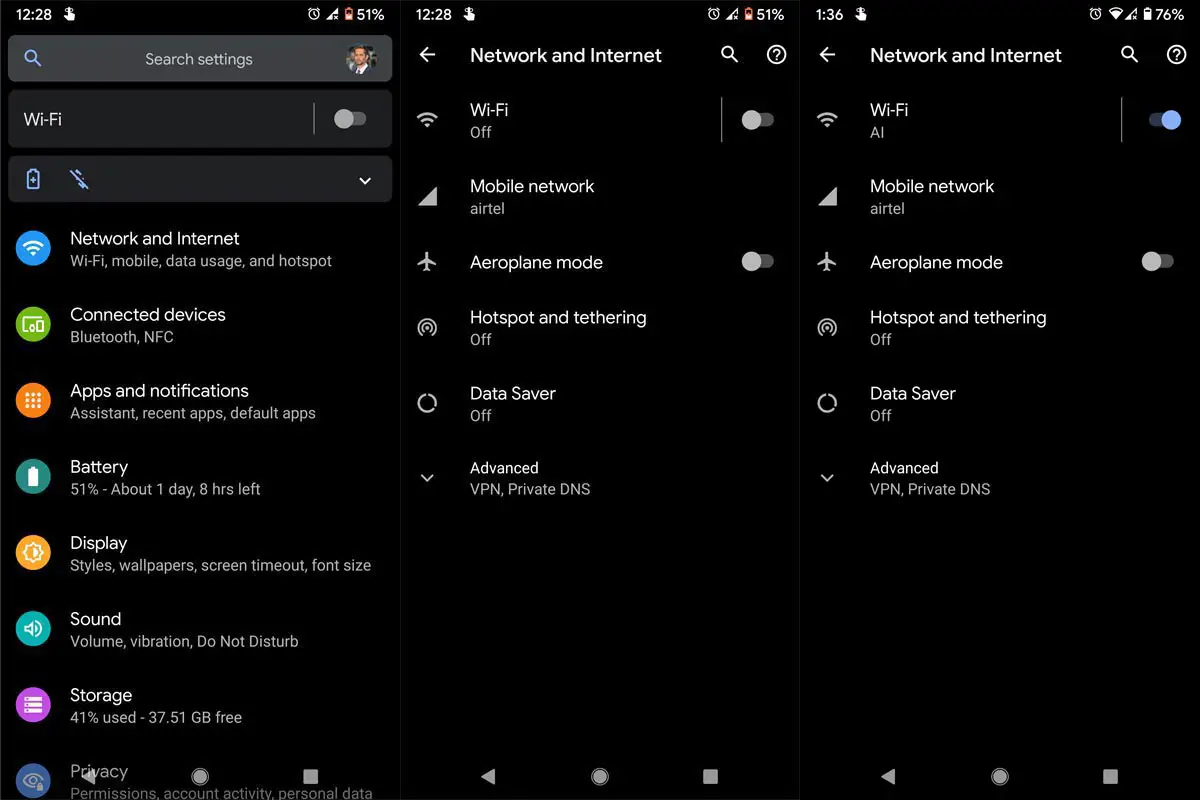The image features a screenshot divided into three distinct columns against a black background. 

**Left Column:**
- **Time:** "12:28"
- **Battery:** "51%"
- **Search Box:** A dark gray box with a blue magnifying glass icon and white text.
- **Options:**
  - **Search Engines**
  - **Search Settings**
  - **Wi-Fi**
- **Battery Icon:** Blue in color.
- **Connectivity:**
  - **Working Internet**
  - **Wi-Fi, Mobile Data Usage, Hotspot**
  - **Connected Devices:** Bluetooth, NFC
- **Apps and Notifications:**
  - **Assistant**
  - **Recent Apps**
  - **Default Apps**
- **Battery Status:** "51% - about one day, eight hours left"
- **Display Settings:** Styles, Wallpapers, Screen Timeout, Font Size
- **Sound Settings:** Volume, Vibration, Do Not Disturb
- **Storage:** "41% used - 37.51 GB FREE"
- **Privacy Settings**

**Center Column:**
- **Time:** "12:28"
- **Navigation Arrow:** Pointing to the left.
- **Network and Internet:**
  - **Wi-Fi:** Off
  - **Mobile Network:** Airtel
  - **Aeroplane Mode**
  - **Hotspot and Tethering:** Off
  - **Data Saver:** Off
  - **Advanced:** VPN, Private DNS

**Right Column:**
- **Time:** "1:36"
- **Battery:** "76%"
- **Network and Internet:**
  - **Wi-Fi:** LL
  - **Mobile Network:** Airtel
  - **Aeroplane Mode**
  - **Hotspot and Tethering:** Off
  - **Data Saver:** Off
  - **Advanced:** VPN, Private DNS

This detailed visualization of settings across three distinct columns appears to be from a digital device's settings page, possibly displaying various connectivity and configuration options in a structured format.